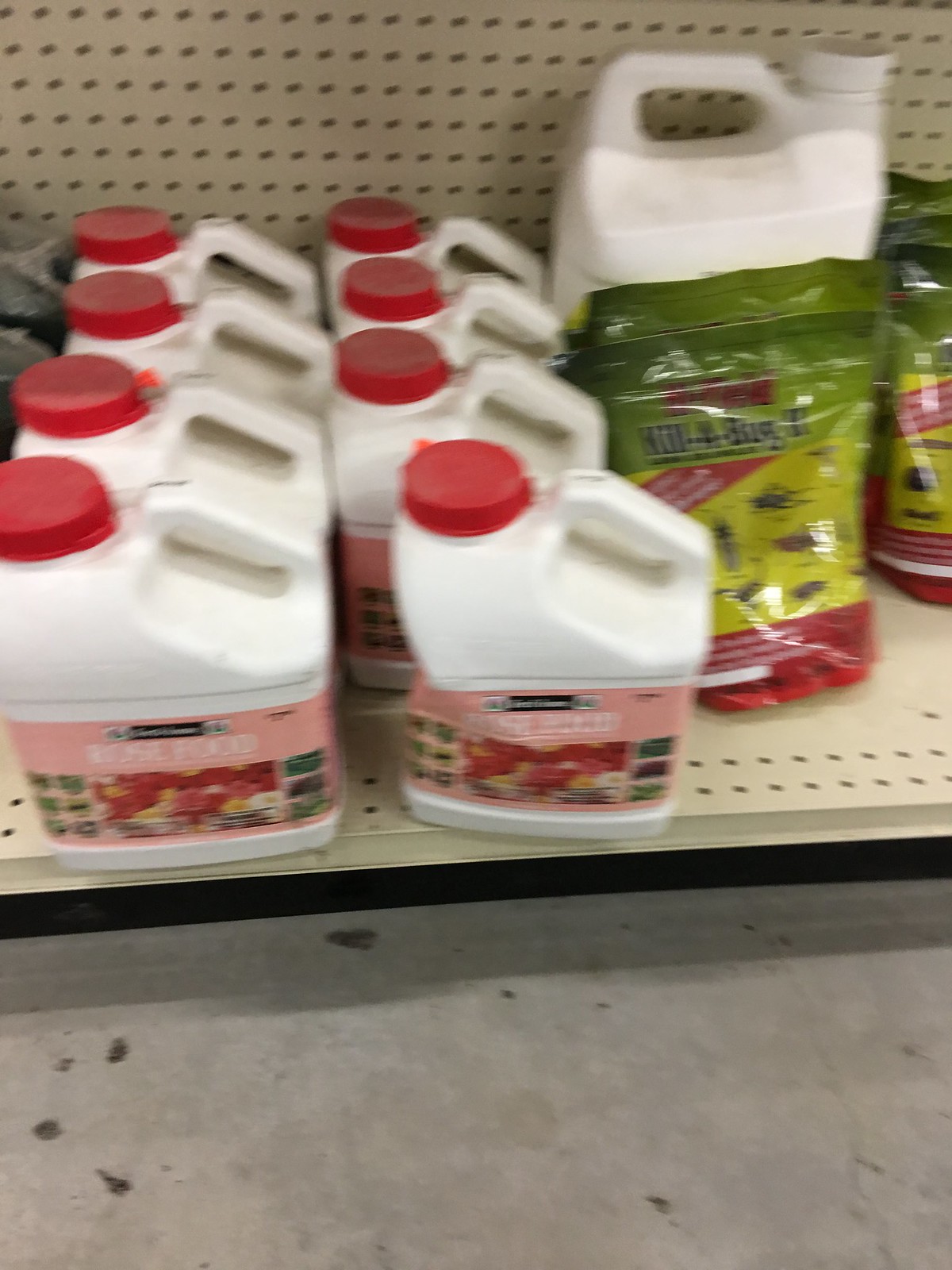This photograph, taken inside a garden center shop, captures a scene filled with a sense of functionality amid the somewhat disordered backdrop. Despite its blurry and low-quality nature, the image clearly shows a white metal shelf positioned close to the grey, concrete-style floor. The shelf is adorned with eight large, gallon-sized bottles, all uniform in their white color with red lids. The labels on these bottles, though unclear, bear the words "Rose Food" along with an image of flowers, suggesting their purpose as plant nourishment. Adjacent to these bottles rests a plastic packet emblazoned with the text "Kill-a-Bug" and accompanied by illustrations of various insects. The background of the shop is perforated with an array of holes, adding to the industrial and utilitarian feel of the setting. This snapshot, likely from a garden center, depicts a humble yet essential corner of gardening supplies.